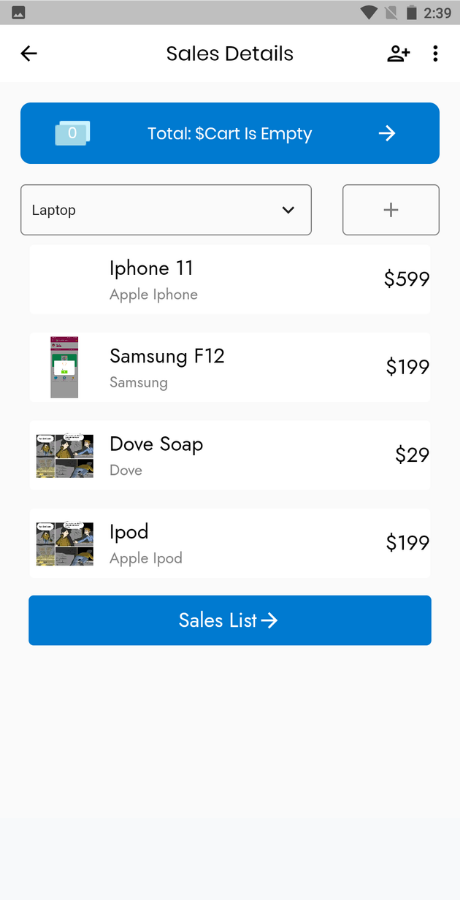Screenshot of a smartphone interface displaying sales details. The background is white with a very light gray header at the top. The time is shown at 2:39 on the right side of the header, alongside a battery icon indicating near-full charge and a Wi-Fi symbol. Beneath the header, the main title "Sales Details" is presented in gray font.

In the upper right corner, there's a user account icon depicted as a circle above a larger semi-circle. Below this, a rectangular button with rounded corners in turquoise blue features the white text "Total S-Cart is Empty."

Below the button, a list of items is shown in gray font:
- iPhone 11 - $599
- Samsung F12 - $199
- Dove Soap - $29
- iPod - $199

At the very bottom, another rectangular button with rounded corners in blue displays the text "Sales List" in white, accompanied by a right-pointing arrow.